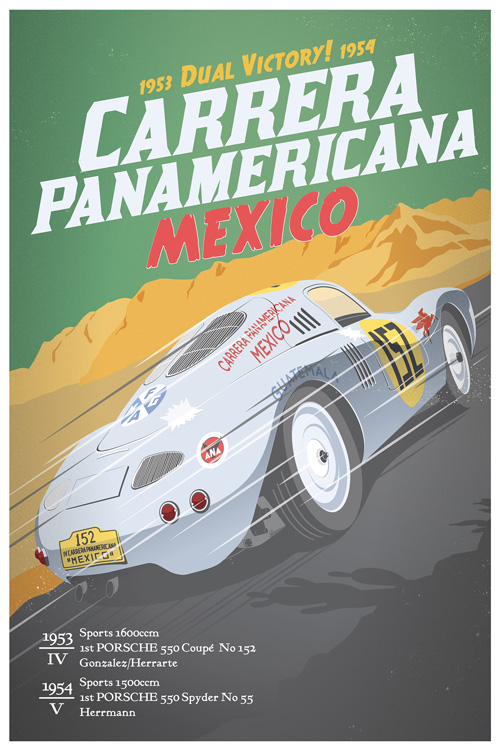This artwork appears to be a vibrant illustration celebrating the Carrera Panamericana races of 1953 and 1954. At the top, set against a green background, the years "1953" and "1954" are emblazoned in yellow with the phrase "Dual Victory!" Between the years, bold white letters announce "Carrera Panamericana," while "Mexico" is highlighted in red beneath. Majestic gold-colored mountains fill the backdrop, framing a sleek gray race car speeding along a black track.

The race car, featuring the rear license plate "152 Mexico," is decorated with various inscriptions including "Carrera Panamericana" and "Mexico" on its sides. A prominent yellow circle on the passenger door displays the number "152," while the front of the car boasts an emblem of a red horse with wings.

At the bottom of the artwork, detailed achievements of the races are highlighted. For 1953, the text reads: "Sports, 1600 CCM, First Porsche 550 Coupe, Number 152, Gonzales, Harate." For 1954, it states: "Sports, 1500 CCM, First Porsche 550 Spyder, Number 55, Herrmann." These inscriptions are presented alongside Roman numerals IV for 1953 and V for 1954, honoring the sequence of the events.